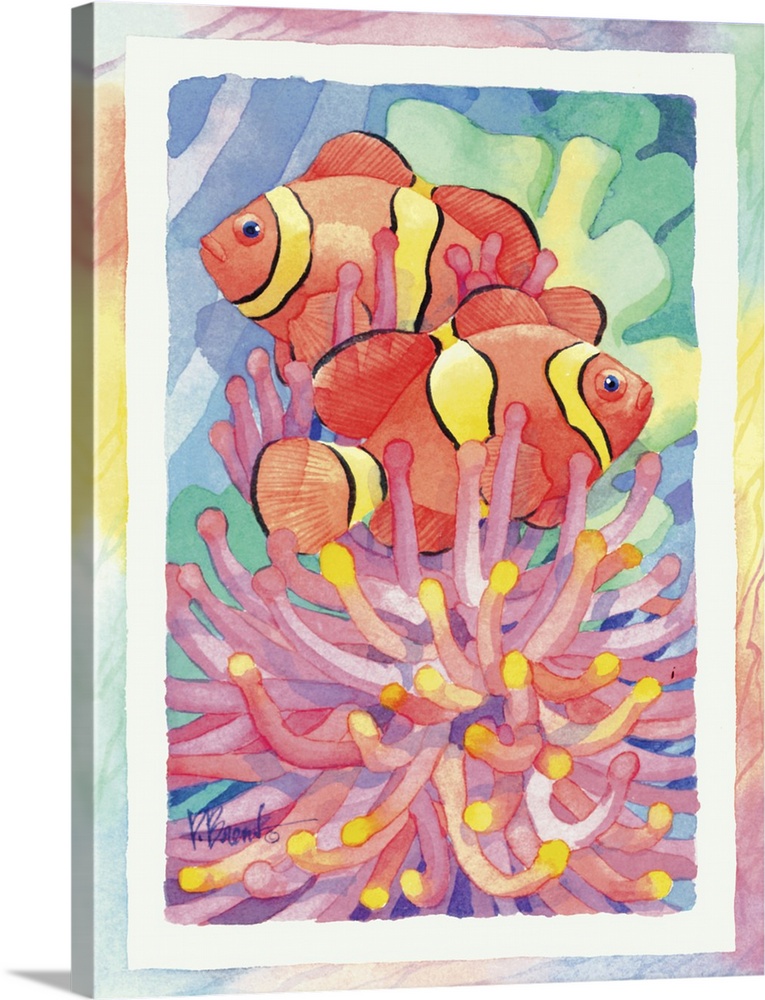This detailed painting showcases two vibrant clownfish nestled amidst the colorful tendrils of a sea anemone at the ocean's bottom, emitting a sense of a natural underwater haven. Encircled by a strikingly rainbow-colored frame that features abstract brush strokes in hues of yellow, blue, purple, and green, the artwork is further divided by a white border that enhances its vivid essence. The clownfish, with their characteristic orange bodies adorned by distinct vertical yellow stripes trimmed in black, are swimming in opposite directions—one to the left and the other to the right. Their habitat, a vibrant sea anemone, exhibits shades of pink, purple, blue, and yellow, providing both a visual feast and a natural shield for the fish. The background reveals additional coral patches in green and yellow tones, contributing to the depth and complexity of the scene. Notably, the canvas is slightly skewed to one side, and a signature, possibly reading "P. Brent," adorns the lower left-hand corner, adding an authentic touch to this captivating marine depiction.